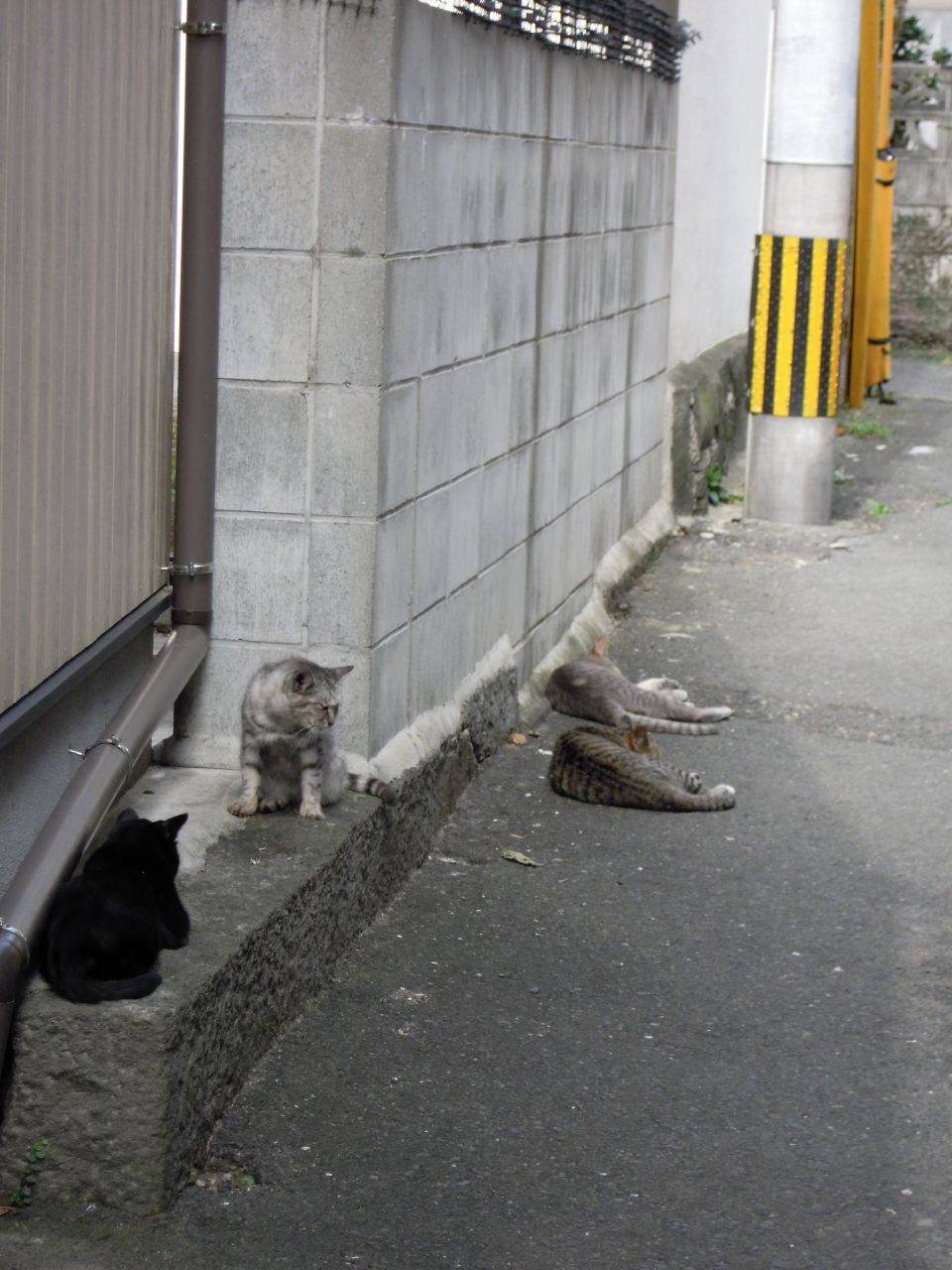This colored photograph captures a bleak urban alleyway scene dominated by four cats. To the left, a black cat, seen from behind, has its tail or possibly a pipe curving downward, obscuring its face. Foreground and slightly to the right is a light gray and white striped tabby, attentively looking off to the right. Centered and lying on their sides against a light gray cinder block wall are two more gray tabby cats. They appear motionless, likely resting on the rough, gray asphalt paving that stretches across the image. The setting is drab, bordered by a darker gray retaining wall on the left and a backdrop that includes a cement block building. A yellow and black striped pipe, or possibly a sleeve-covered pole, adds a splash of color to the otherwise somber environment. A brown drainage pipe is also visible, contributing to the utilitarian and stark surroundings. The overall atmosphere is one of urban desolation, with more street and structural elements than greenery or warmth.